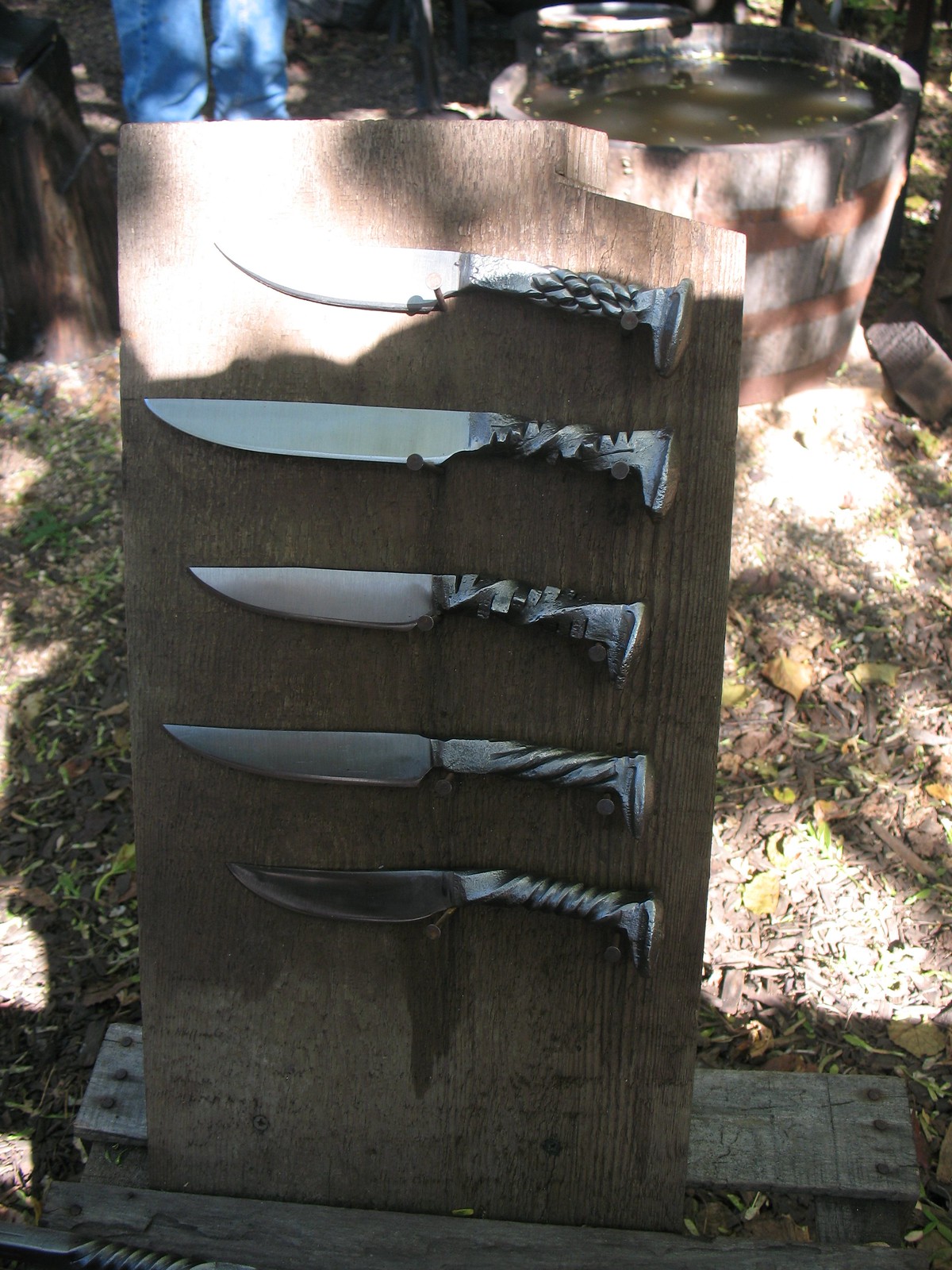This color photograph captures a set of five intricately designed knives displayed horizontally on a vertical wooden board. These knives, likely made of silver or steel, feature blades with various curved shapes and are embellished with decorative handles. Some handles exhibit twisted designs, while others appear to have etched patterns. The board they rest on is a vertical, thin rectangular piece of wood, supported at the bottom by a horizontal plank. Sunlight delicately highlights the blades, particularly illuminating the first knife and the right side of the background. The ground in the backdrop appears greyish with small patches of budding foliage, indicative of early spring. In the upper right-hand corner, a round wooden object with three horizontal red stripes is visible. Additionally, a partially obscured blue object is detectable in the upper left corner, just above the wooden plank. This meticulously arranged outdoor setting provides a rustic and intriguing visual composition.